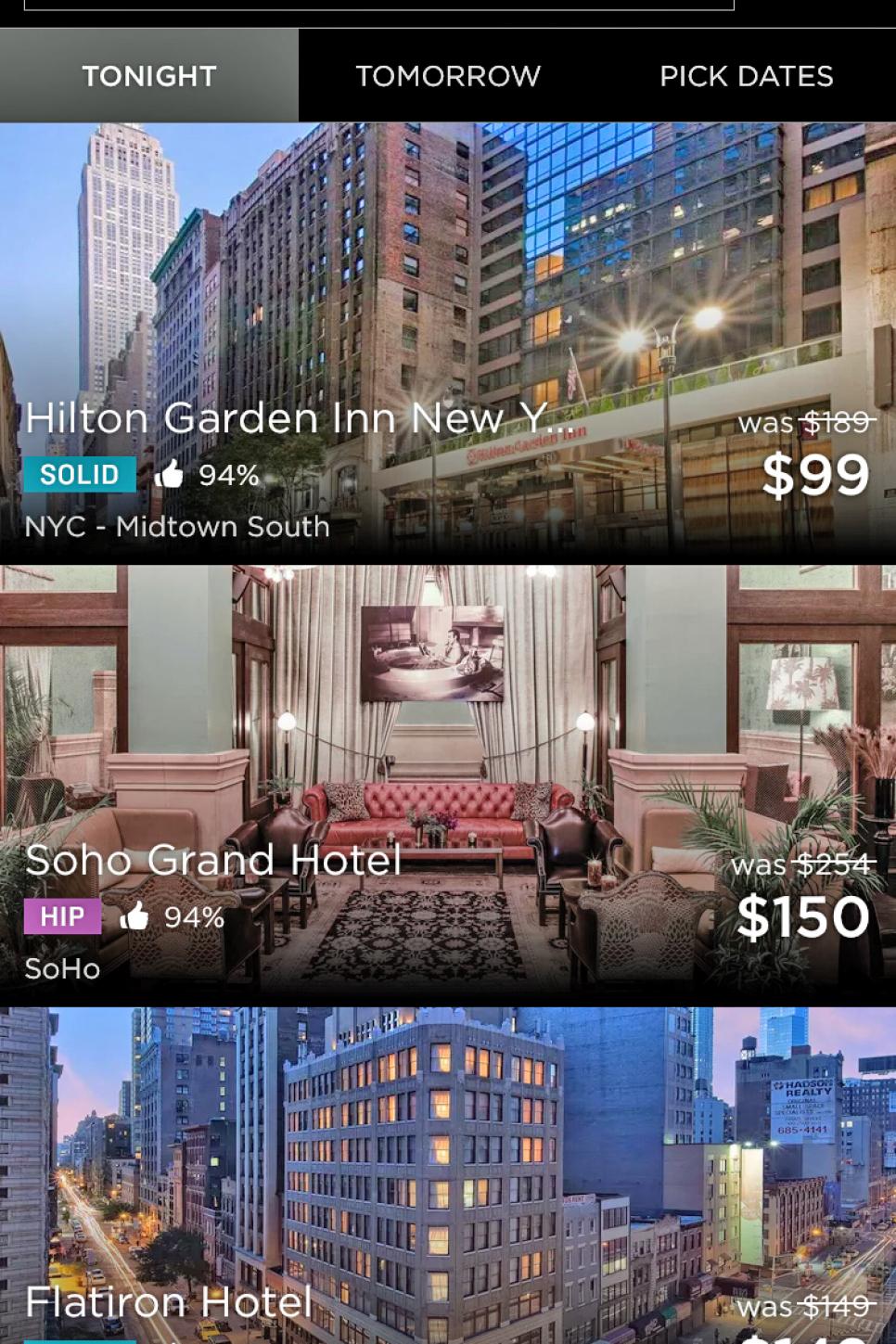Screenshot displaying three hotel options, with visuals of their buildings, special offers, and ratings:

1. **Hilden Garden in New York**: Featuring an exterior shot of the towering building with glassy windows. Originally priced at $189, it’s on sale for $99. Located in NYC Midtown South, it boasts a solid 94% thumbs-up rating.
  
2. **Soho Grand Hotel**: Showcasing a particularly lavish room. Initially $254, now available for $150. Situated in Soho, it has a "HIP" label signifying its trendy appeal.
  
3. **Flat Iron Hotel**: Depicts the building's exterior on a corner, resembling an office structure. Was priced at $149, though the current price is not visible. This hotel combines unique architecture with a prime location.